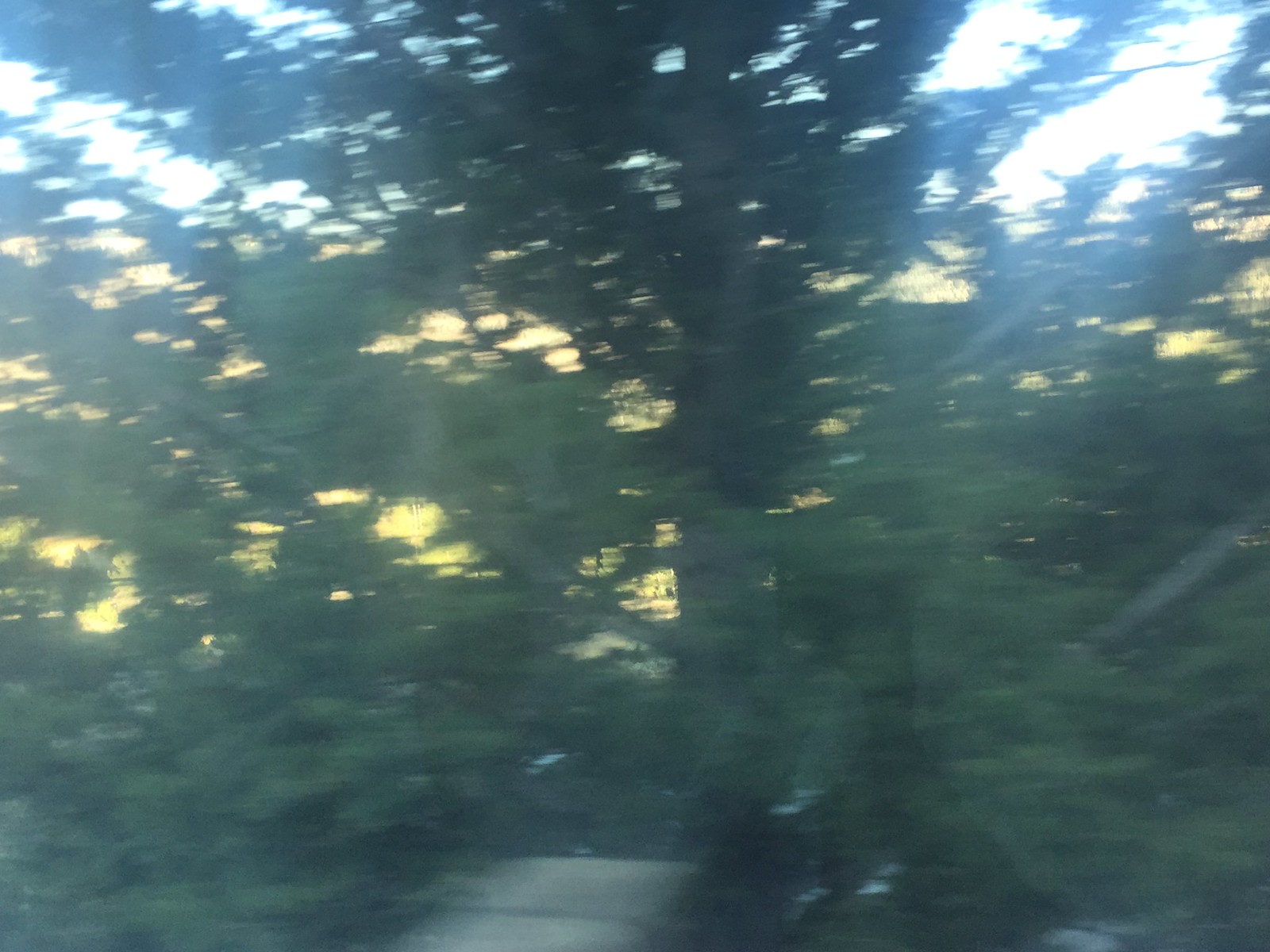A blurry photograph captures an evergreen tree from beneath its shadowed canopy. The thick branches obscure a view of sunlit foliage and a bright sky in the background. Motion blur and light bleed contribute to the muddied quality of the image, with predominant colors being dark greens, mid-tone greens, light greens, white, and black. At the very bottom center, a potential stone walkway or path points towards the tree, though the blur makes it hard to distinguish its precise details.